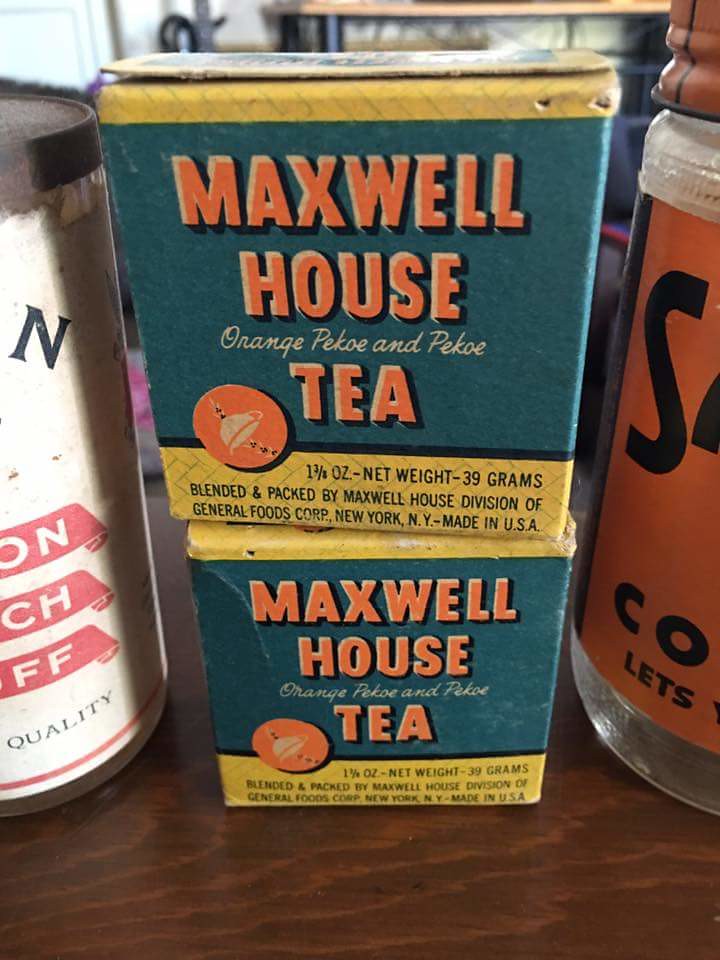In this image, various items are arranged on a brown wooden table. The most prominent item is an old, possibly ancient, box of Maxwell House Orange Pekoe and Pekoe Tea. The box features the brand name "Maxwell House" in large orange bubble letters. It indicates a net weight of 1 and 2/8 ounces, equivalent to 39 grams. The tea is blended and packed by the Maxwell House Division of General Foods Corp, located in New York, New York, and was made in the USA. Beside the tea box, there is a white jar with a large white label. The bottom of the label features the word "quality." The items together suggest a sense of nostalgia and a glimpse into product packaging from the past.